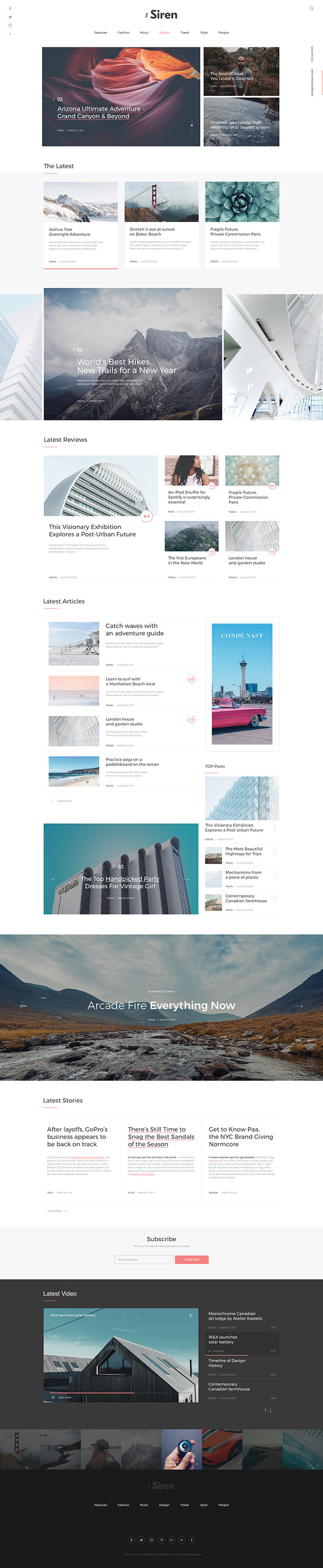**Website Interface Overview for "Siren"**

The webpage titled "Siren" features a sleek and minimalist design, predominantly in a monochromatic color scheme with strategic splashes of vibrant hues. Here's a detailed breakdown of its layout:

**Header Section**
- The title "Siren" is prominently displayed at the top center of the page in white text against a black background. The name is spelled out as "S-I-R-E-N."
- On the far left, there are small white buttons featuring grey symbols representing popular social media platforms: Facebook, Twitter, Instagram, and an additional 'plus' icon for more options.

**Navigation Bar**
- Centrally positioned beneath the header, there are several white buttons with black text:
  - Features
  - Fashions
  - Music
  - Design (highlighted in red, indicating it is currently selected)
  - Travel
  - Style
  - People

**Main Content Area**
- Below the navigation bar, a striking visual showcases a blend of vibrant sand dunes in hues of red, maroon, purple, and orange.
- On the left side, the text "O2 Arizona Ultimate Adventure - Grand Canyon and Beyond" is displayed in white.

**Featured Articles**
1. **First Article**
   - On the right side, a photograph depicts an African American individual seated in a clearing near trees with a darkened grey sky. The individual is wearing a grey short-sleeved t-shirt and black pants, arms crossed, showcasing a muscular build.
   - The caption reads: "This Sound Cloud You Loved Is Doomed."
   
2. **Second Article**
   - An image from space showing Earth, referred to as a blue marble with white clouds.
   - The caption states: "OneWeb Vouches for High Reliability of its DeOrbit System."

3. **Latest Articles**
   - A snowy mountain with grey and rounded peaks, labeled "Joshua Tree Overnight Adventure."
   - An iconic image of the San Francisco Bridge, detailed in its characteristic brown and red colors.
     - Caption: "Stretch It Out at Sunset on Baker Beach."
   - A close-up shot of a blue flower with pointy petals.
     - Caption: "Fragile Future, Private Commissioned Plant for Paris."
   - A towering, dark grey mountain titled "World's Best Hikes, New Trails for New Year."
   - A large white building with extensive windows, accompanied by a skyscraper with an arched top.
     - Caption: "Visionary Expedition Explores the Post-Urban Future."
     - Along with a red open circle featuring the number "6.4."

4. **Additional Imagery**
   - Miscellaneous pictures towards the page's lower section, including:
     - A large grey building.
     - A scenic stance showing mountains on either side, colored in grey and orange, leading up to what appears to be a frozen lake.
     - Caption: "Arcade Fire, Everything Now" in bold white text.

This organized structure allows users to navigate through various sections, giving a comprehensive visual and textual summary of the webpage’s content.